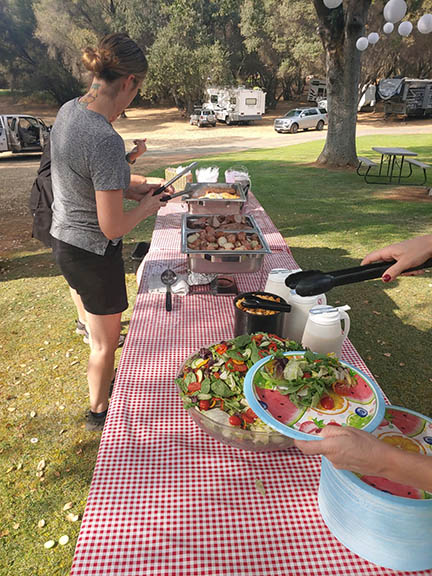In this realistic, vertically oriented photograph taken outdoors on a sunny day, we see a charming picnic setting likely situated in a park or campground area. The foreground is dominated by two or three picnic tables covered with a red and white gingham tablecloth, arranged in a line and laden with a delicious array of food. A prominent feature at the center is a bountiful salad bowl surrounded by various chafing dishes filled with mashed potatoes and other delectable items. Paper plates adorned with watermelon patterns and a blue stripe line the tables.

Two figures are engaging with the spread: on the left, a woman with red hair tied up in a bun, wearing a gray T-shirt and black shorts, is seen from behind as she helps herself to some food. On the right, only the hands of another person are visible, holding tongs and a paper plate while serving some salad.

In the background, the scene expands to show green grass, several trees, and a myriad of vehicles including white and gray RVs and cars. Additionally, a picnic table stands beside a tree on the far right, and white balloons dangle from the branches, adding a festive touch to the serene setting. This beautifully captures the essence of a relaxed outdoor gathering amidst nature and parked RVs.